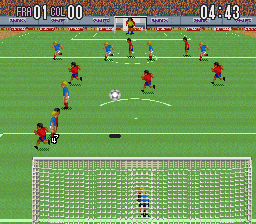This screenshot captures a nostalgic moment from a classic 8-bit video game, vividly illustrating a pixelated soccer match. The scene is viewed from the perspective of the goalie, who is centrally positioned in front of the goal. The goalie is poised to intercept a ball coming towards his left-hand side. The players are distinguishable by their jerseys—the team in red plays against opponents in green. The scoreboard on the top left corner indicates the current score as 1-0. The top right corner shows the timer, displaying 04:43, likely indicating the remaining time in the halftime segment of the match. The pixelated art style and gameplay elements evoke a strong sense of retro gaming nostalgia.